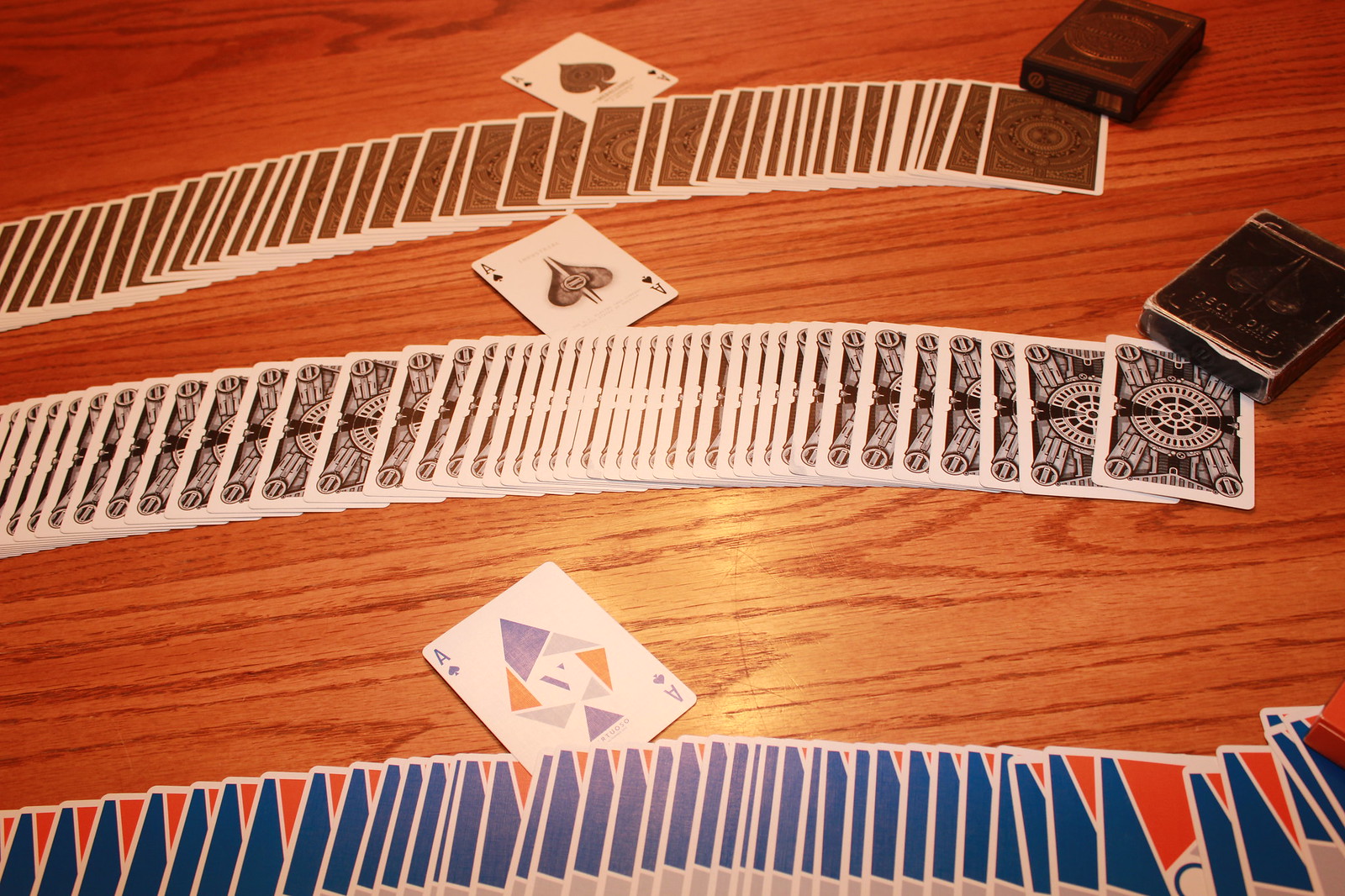An indoor color photograph taken from an angled, above perspective shows a dark brown wooden table or countertop. Displayed on the surface are three fanned-out decks of playing cards, each with distinct back designs, arranged in horizontal rows.

At the top, the first row of cards stretches almost completely from the left edge to the right. In the upper right corner of this row, a card box rests on the very last card, oriented diagonally at a 45-degree angle. Centrally within the row, the Ace of Spades is prominently visible, angled with its top pointing to the upper left and bottom to the lower right.

The middle row mirrors the arrangement of the top row, with a sequence of fanned-out cards starting from the left and extending almost to the right edge. Similarly, the deck’s box is placed diagonally over the last card on the right. The Ace of Spades in this row is also face-up and aligned in the same diagonal orientation as the one above.

At the bottom, a third row of cards follows the same pattern. However, this row is partially cut off by the lower edge of the photograph, so only part of the cards is visible. Despite this occlusion, it is evident that the cards fan out from the lower left to the right, with just the corner of the card box peeking from the right side. The Ace of Spades from this deck is oriented identically to the aces in the rows above, with its top pointing to the upper left and bottom to the lower right.